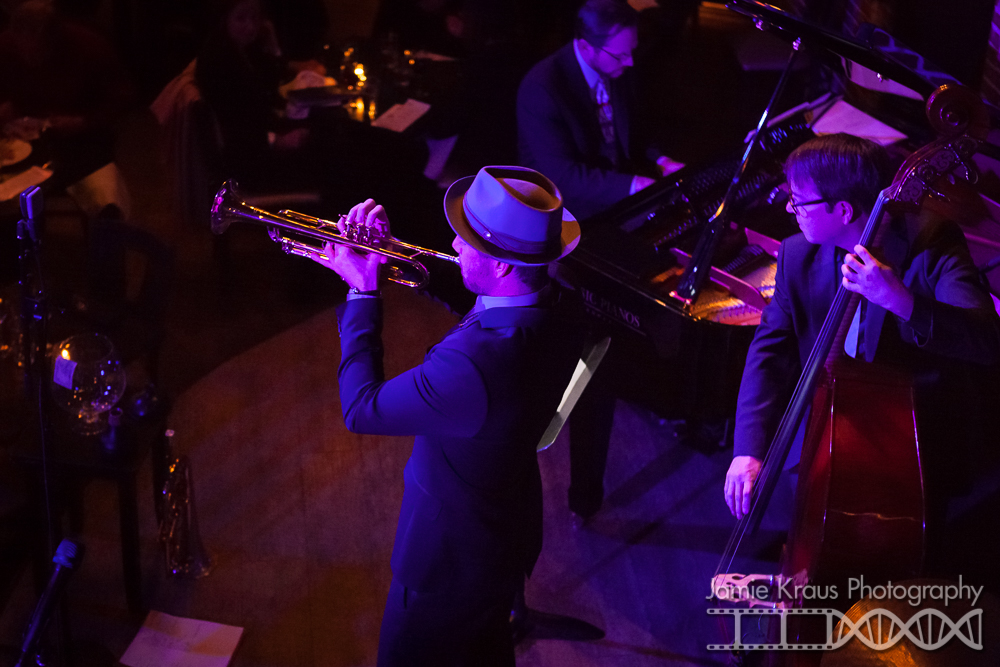An overhead view captures a jazz band performing on stage in a dimly lit club, bathed in a soft purple and bluish light. The elegance of the scene is accentuated by the musicians' attire; all three are dressed in dark suits with ties, exuding a classic and sophisticated look. The frontman, distinguished by his navy blue or dark suit and a fedora, commands attention as he plays a brass trumpet. Behind him, another musician skillfully handles an upright bass, providing the rhythmic backbone of the ensemble. At the black grand piano, the third member complements the tune with intricate melodies. The intimate club setting features a few tables with what appears to be candlelight, where patrons are likely enjoying the immersive jazz experience. The photograph, taken by Jamie Krause Photography, captures not only the musicians but also the ambiance of the cozy venue.